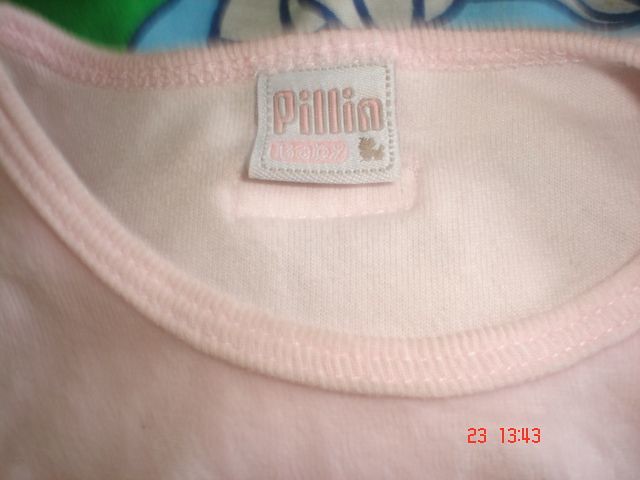This is an up-close photograph of a pink child's shirt, showcasing the tag sewn into the neckline. The tag is square and white with pink font reading "PILLIN," and underneath in a pale pink font, it says "baby." To the right of the text, there is a small brown character, which appears to be an animal, possibly a dog or a chicken. The shirt features faint white pink stitching around the collar and back of the neckline. Behind the shirt, there is a soft material in shades of green, light blue, blue, and white, with some areas outlined in black. At the bottom of the image, red numbers read "23 13..43."